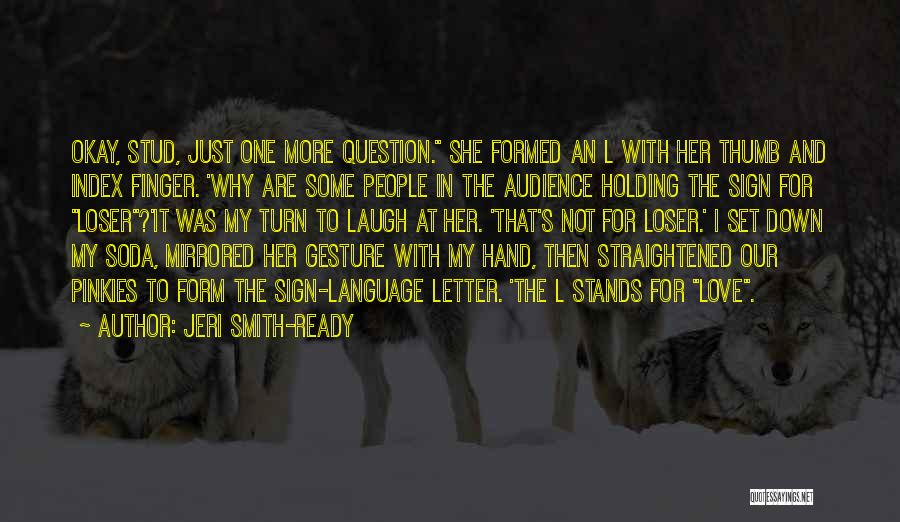The image is a meme-like quote set against a wintery forest backdrop with four wolves in the snow. The wolves are somewhat muted and not the main focus; two are lying down on the outer edges, facing the camera, while the two in the center are standing, one angled left and the other facing the camera but obscured by text. The setting is a snow-covered clearing with dark, leafless trees, indicative of winter. Overlaid in bold yellow capital letters, the quote reads, "Okay, stud, just one more question. She formed an L with her thumb and index finger. 'Why are some people in the audience holding the sign for loser?' It was my turn to laugh at her. 'That's not for loser.' I set down my soda, mirrored her gesture with my hand, then straightened our pinkies to form the sign language letter. The L stands for love." The quote is attributed to author Jerry Smith-Ready. In the bottom right corner, a white rectangle with black text reads "quotesayings.net".